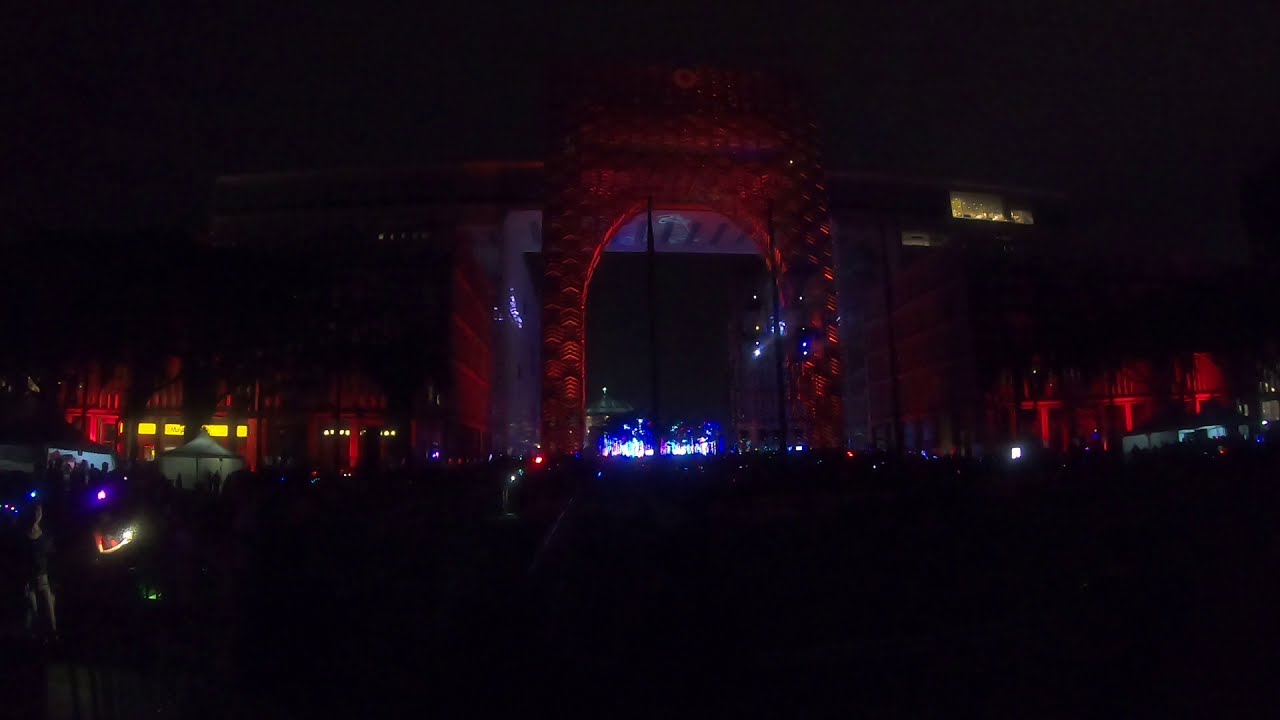The image captures a dark night view of a building's front exterior, primarily illuminated by red spotlights that obscure much of its architectural details. Centered in the building, there is a large archway, through which an array of LED and spotlights can be seen, enhancing the scene's dramatic lighting. The sky above is pitch black, adding to the overall dark ambiance. To the left side of the image, a white tent emits light from within, casting various shadows of people inside, suggesting activity. Additional tents are also positioned to the right in front of the building, similarly lit from inside with visible shadows of occupants. The absence of streetlights and the concentration of lighting within and through the arch create an enigmatic atmosphere that hints at a significant event or gathering, possibly a concert or a public spectacle. Despite the darkness and the vague outline of people or objects in the foreground, the photo emphasizes the vibrant, albeit obscured, nighttime energy of the scene.